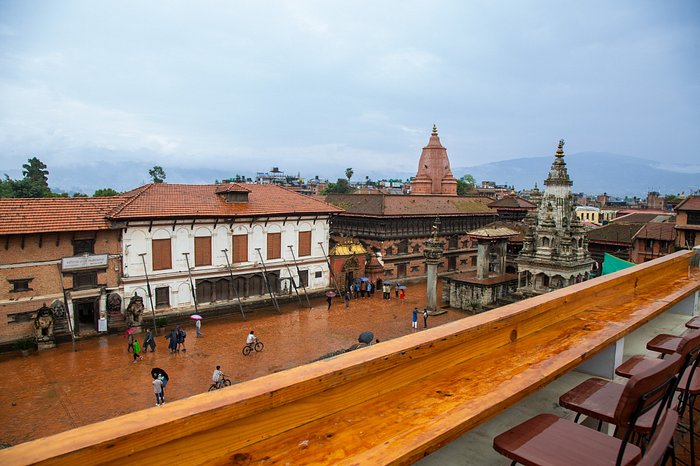The photograph captures a detailed urban scene from a balcony, possibly part of a rooftop bar or restaurant. The balcony features multiple brown chairs facing outward toward a view framed by a solid, wet wooden railing, indicating a rainy day. The sky is dark gray, casting a somber tone over the scene. Below, a busy street comes to life with many people walking and riding bikes, some holding umbrellas against the rain. This street appears to be part of a piazza or large courtyard, richly decorated with statues and other ornaments. 

In the distance, faint outlines of mountains emerge through the hazy backdrop. The buildings lining the far side of the street exhibit a Western European architectural style, characterized by white walls and brown brick walls, with the nearest building showing bricked-up windows. These buildings possess red ceramic-tiled roofs, adding a touch of color to the scene. Notably, an old, stone structure with a pointed top—possibly a religious temple—stands prominently, suggesting the photograph might be taken in a Southeast Asian city known for its mix of historical and cultural architecture. The historical ambiance is further enhanced by the weathered appearance of the stone structure and the overall historical aesthetics of the surroundings.